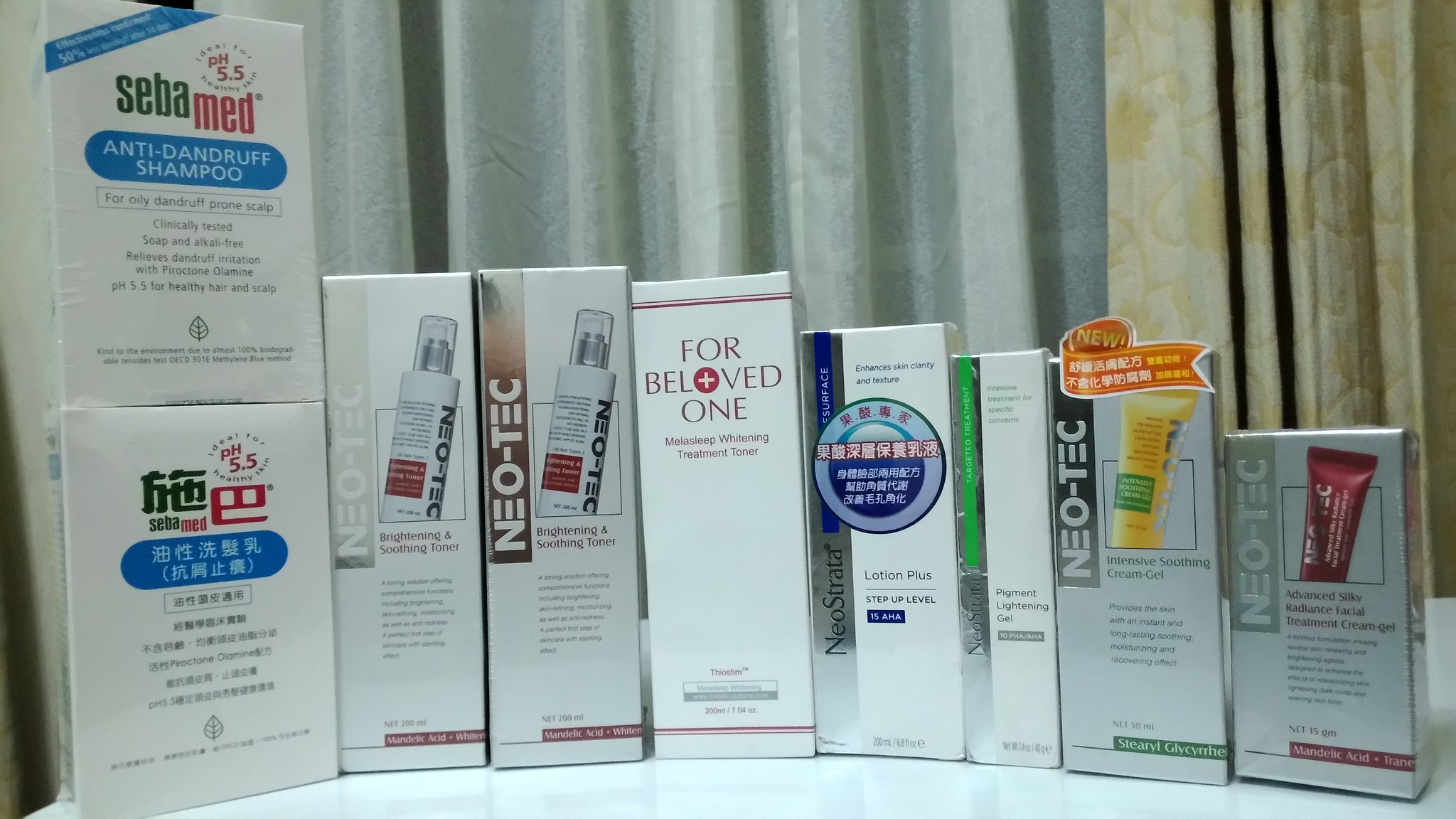The image appears to be an advertisement for the brand Neotech, showcasing a range of their products displayed on a pristine white table. In the background, the setting includes a combination of cream-colored see-through curtains and a darker cream or yellow cotton curtain, adding a soft, elegant touch to the scene. On the table, there are ten product boxes arranged in an orderly fashion.

On the right side of the table, there are two gray boxes featuring the Neotech branding, one of which includes the phrase "For Beloved One." Alongside these, there are five white boxes also under the Neotech brand. The precise nature of the Neotech products isn't entirely clear, but they appear to be lotions or shampoos.

Moving to the left side of the table, there is a stack of two boxes. The top box is an anti-dandruff shampoo by the brand Seba Med. It sits on what seems to be another box, possibly just the reverse side of the same shampoo box, which displays text in Japanese. Though the details of the Japanese writing are unclear, the Seba Med branding is visible.

Overall, the image is a clean, organized presentation of various Neotech products, complemented by a single Seba Med item, set against an aesthetically pleasing backdrop.